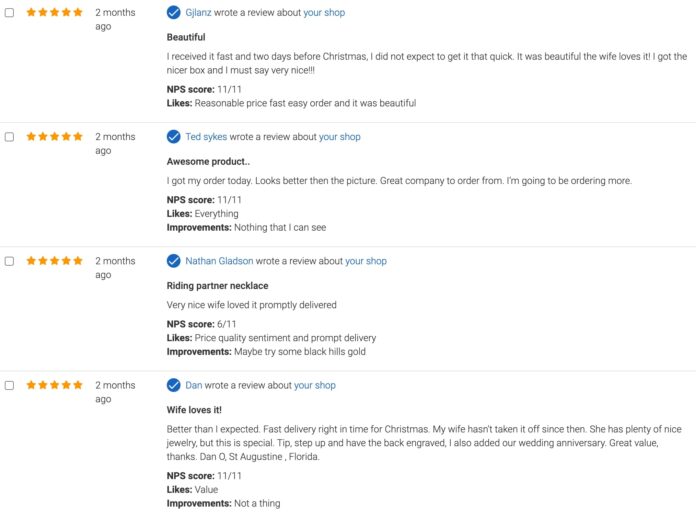This screenshot captures a reviews page from an unspecified online shop, possibly selling jewelry given the nature of the feedback. There are four five-star reviews, all dated from two months ago, each by a different reviewer.

1. **Reviewer: Jalons**
   - **Rating:** ★★★★★
   - **Review:** Jalons expresses his surprise and satisfaction in receiving his order two days before Christmas, much earlier than expected. 
   - **Commentary:** The prompt delivery exceeded his expectations.

2. **Reviewer: Ted Sykes**
   - **Rating:** ★★★★★
   - **Review:** Ted praises the shop for delivering an item that looks even better in person than in the pictures. He expresses high satisfaction with the company and encourages others to order from them as well.

3. **Reviewer: Nathan Gladson**
   - **Rating:** ★★★★★
   - **Title:** Writing Partner Necklace
   - **Review:** Nathan shares that the necklace was very nice, his wife loved it, and it was delivered promptly.
   - **Commentary:** The review highlights both the quality of the product and the swift delivery.

4. **Reviewer: Dan**
   - **Rating:** ★★★★★
   - **Title:** Wife Loves It
   - **Review:** Dan is enthusiastic about the purchase, noting that the item exceeded his expectations. It arrived just in time for Christmas, and his wife, despite owning plenty of nice jewelry, finds this piece special and hasn't taken it off since then.

The consistent mention of fast deliveries, particularly before Christmas, and the repeated satisfaction with the products suggest a reliable and potentially well-liked online jewelry shop.